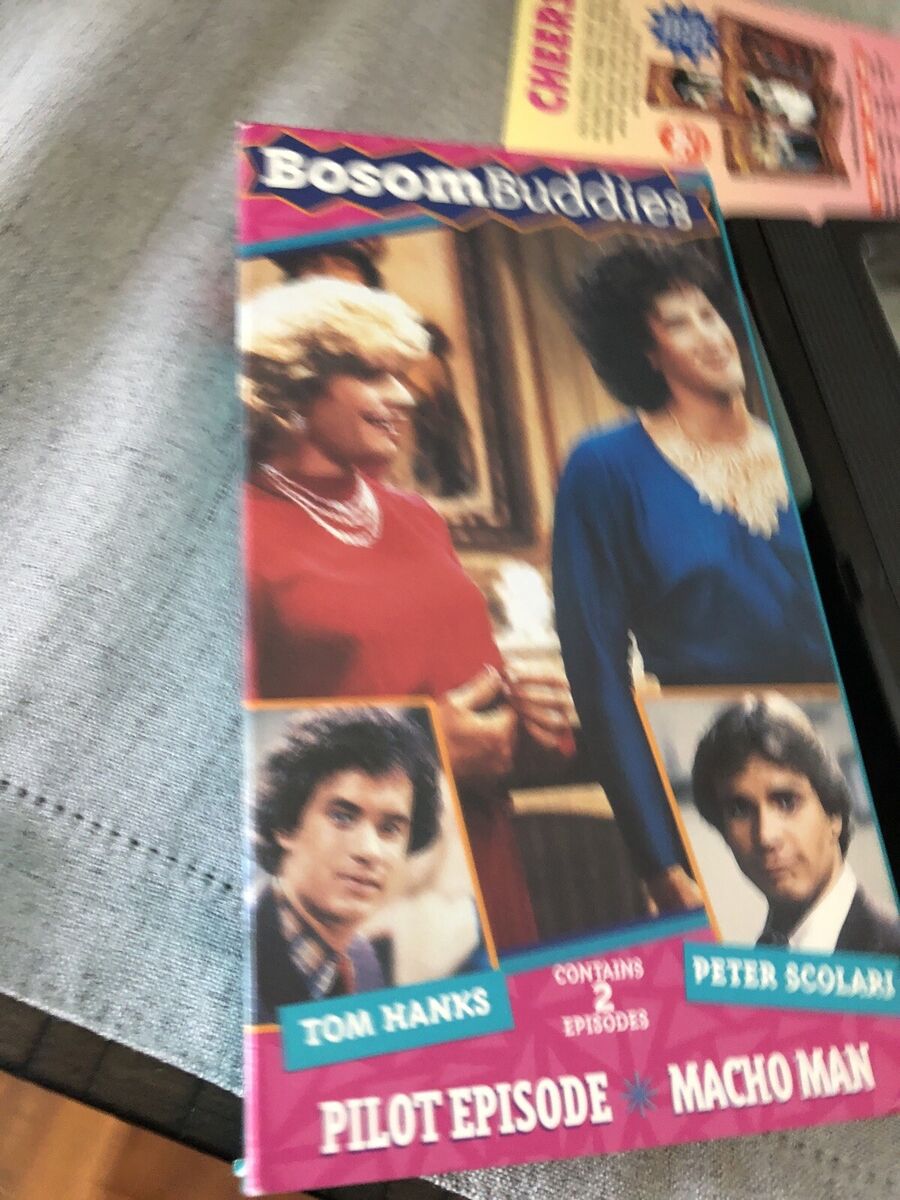This image captures a VHS case for the TV show "Bosom Buddies," featuring Tom Hanks and Peter Scolari prominently on the cover. The case displays a large, somewhat blurred photo, set against a backdrop of gray fabric with hints of brown hardwood. Both actors are depicted twice on the cover: dressed in their series character costumes (Hanks in a blue long-sleeved shirt with a lace collar and white skirt, and Scolari in a red dress with pearls) and also in their regular appearances within the series. The VHS cover includes text that reads "Bosom Buddies," as well as specific details such as "Contains Two Episodes: Pilot Episode and Macho Man" and the actors' names, Tom Hanks and Peter Scolari. Additionally, part of the actual VHS tape is visible, slightly protruding from the right side of the case. Behind the "Bosom Buddies" VHS, there is another VHS case, this one for the show "Cheers," though it is mostly out of focus apart from the recognizable title.